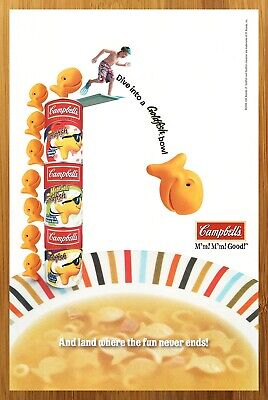The image is a vertically-aligned advertisement framed by a medium brown wood border, resembling a poster. The top portion of the poster features a clean, white background with three stacked Campbell's soup cans, easily recognizable with their iconic red and white labels. Emerging from these cans, a line of goldfish crackers creates a whimsical, ascending ladder leading to a blue diving board. Positioned at the edge of the diving board, a boy—poised to dive—further animates the scene. The text "Dive into a goldfish bowl" dynamically surrounds him, enhancing the playful atmosphere.

On the left, a goldfish wearing sunglasses adds a quirky element as it dives downward along with the boy. At the bottom of the advertisement, a bowl filled with Campbell's soup is depicted, with goldfish crackers floating cheerfully in the broth. Over this bowl, white text reads, "and land where the fun never ends," reinforcing the theme of excitement and enjoyment associated with the product. The color scheme predominantly features white and orange, with accents of yellow and red, capturing attention and tying the promotional elements together visually.